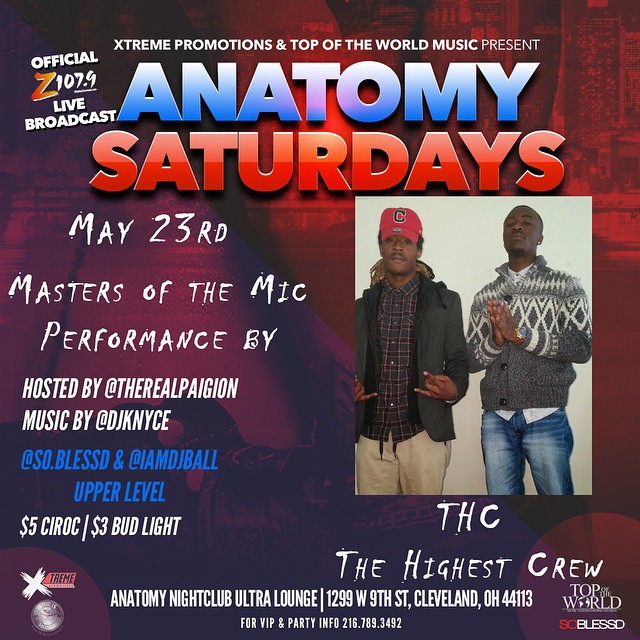The promotional image advertises an event with vibrant red and purple gradients. The top of the image features white text that reads "Extreme Promotions and Top of the World Music Present." Below that, the event's title "Anatomy Saturdays" is prominently displayed, with "May 23rd, Masters of the Mic, Performance by THC, The Highest Crew" in a mix of blue and red fonts. 

An inset photograph on the middle-right shows two African American men posing. The man on the left sports a red baseball cap with a "C," a grey jacket with black lining, a plaid shirt, tan trousers, and he gestures towards the camera. The man on the right wears a grey ski sweater with a Nordic white pattern at the shoulders, a white shirt underneath, and stonewashed blue jeans.

On the upper left corner, tilted slightly upward, is a notice for an "Official Z107.9 Live Broadcast," with the "Z" in red. Below the inset photo, the caption "THC, The Highest Crew" is handwritten in white. The lower section of the image provides event details: "Anatomy Nightclub Ultra Lounge, 1299 West 9th Street, Cleveland, Ohio 44113." For VIP and party info, call 216-789-3482. The left side lists hosts and DJs: "Hosted by @TheRealPageon," and "Music by @DJKnYce, @So.Blessed, and @IAmDJBall." It also mentions "$5 CIROC / $3 Bud Light." The bottom right corner includes the white text "Top of the World" followed by red text "SC" and white text "BLESSED".